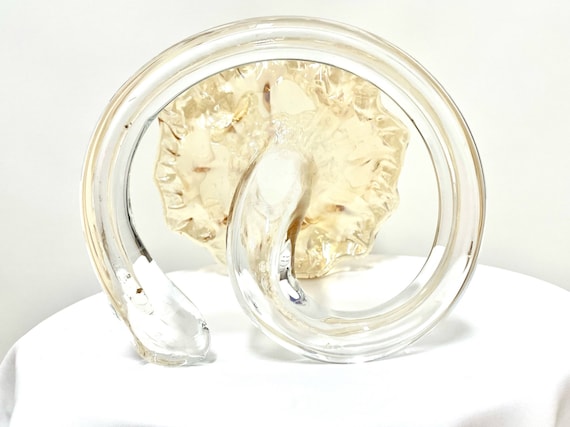The image depicts an artistic glass piece featuring a curved tube forming an almost complete circle, with its open ends turning inward. The tube terminates in a rounded, mushroom-like structure with a brown, beveled appearance, and hints of a metallic, possibly silver, fused embellishment. This delicate creation is positioned on its side atop a table draped in a white cloth, set against a gray background. The unique composition and unconventional design give the impression of a whimsically crafted stem and flower, capturing both organic and surreal elements.